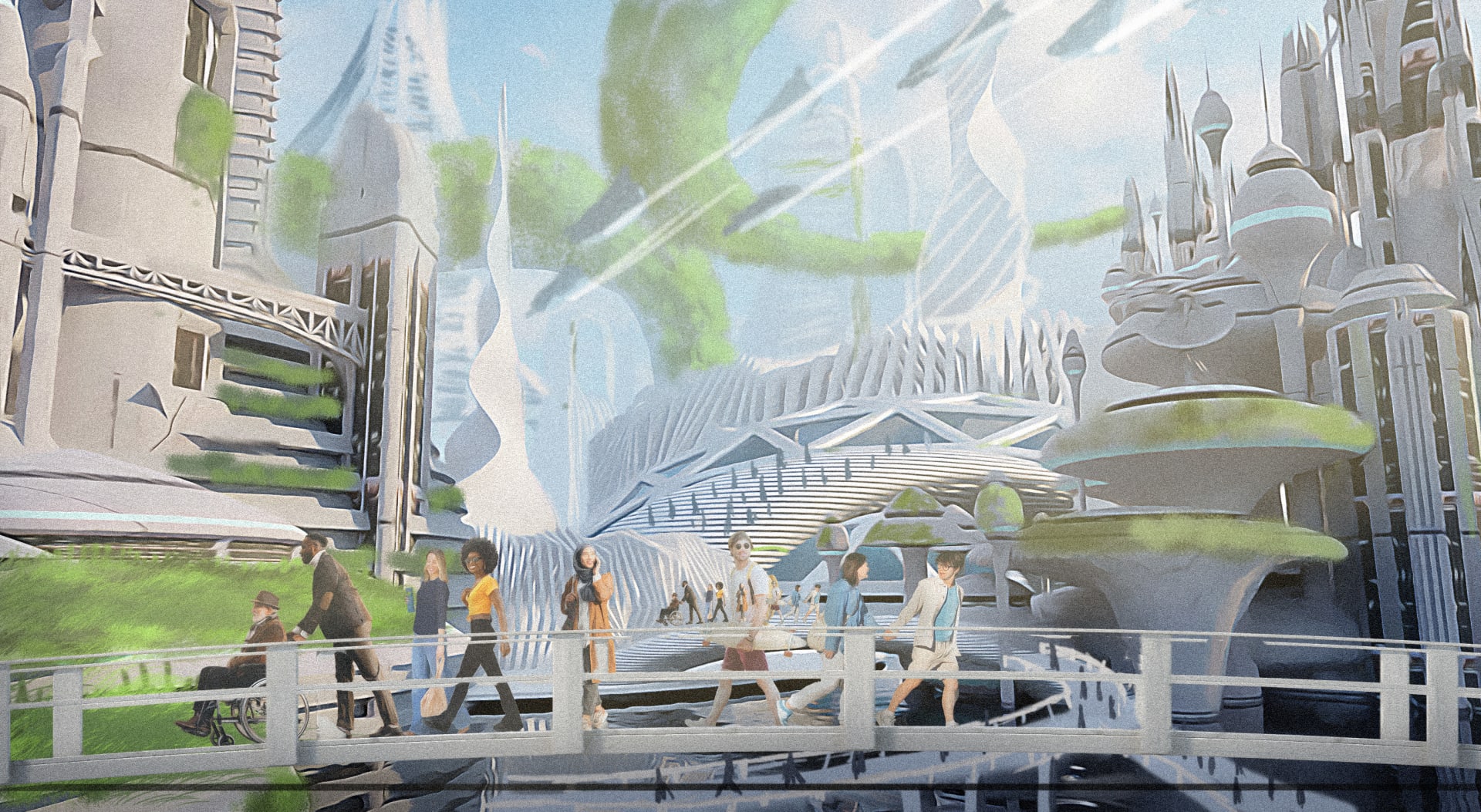This intricate digital art piece portrays a futuristic society, blending lush green landscapes with striking architectural designs. In the background, tall spires and futuristic skyscrapers with needle points and rounded edges rise above the city. Expansive rings of foliage, which could be large trees or greenery, adorn the skyline, adding an element of nature integrated into the urban setting. The cityscape features cylinder-like structures, some covered in moss-like substances, emphasizing a blend of nature and technology.

Moving towards the foreground, three canopies with grass-covered tops emerge from the ground, situated behind a large white arch bridge. The bridge crosses over a body of water, where eight people are depicted walking to various destinations. Among the bridge's pedestrians are a couple holding hands, a man carrying a skateboard and looking towards the viewer, and a woman talking on her phone while gazing over the railing. Additionally, two women, one black and one white, walk together, and a tall black man pushes an elderly white man in a wheelchair. The cityscape and bridge are populated with a diverse array of individuals, suggesting an inclusive and vibrant future society. The overall scene is set against a backdrop of a pale blue sky, creating a vision of a harmonious and advanced future.